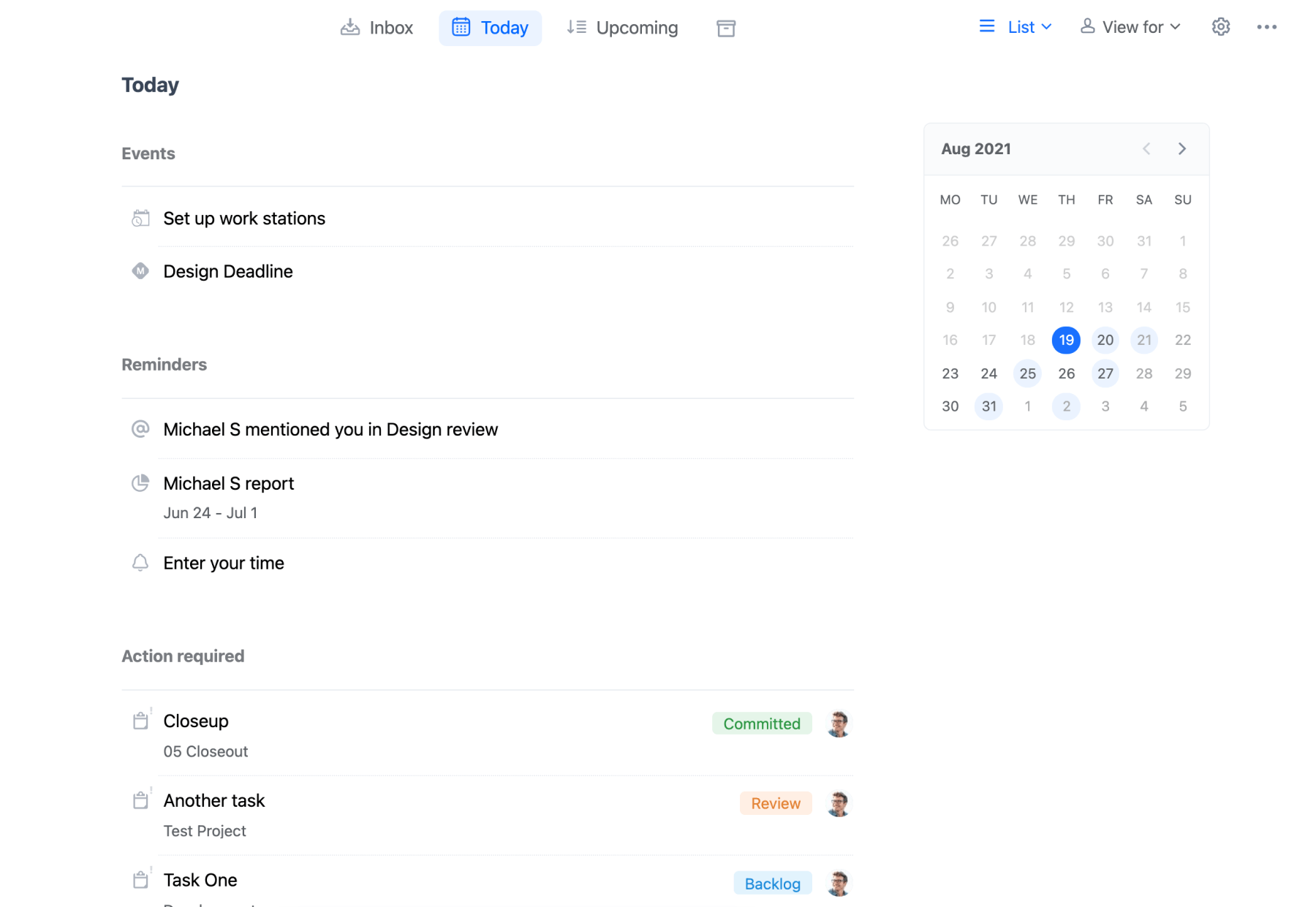The image is a screenshot of a calendar app with a clean, white background. At the top left of the screen, there are three navigational options: "Inbox," "Today," and "Upcoming," with "Today" prominently highlighted in blue. On the upper right, there are three additional options labeled "List," "View For," and "Settings".

Beneath these options, a small calendar is displayed, indicating the month of August 2021. The date August 19th is highlighted in blue, signifying the current day. 

The left section of the screen is headed by the word "Today", followed by a subheading "Events". Listed under "Events" are two items titled "Set Up Workstations" and "Design Deadline." 

The next section, labeled "Reminders," includes notifications such as "Michael S mentioned you in Design Review," "Michael S Report," and "Enter Your Time."

The final section is "Action Required," containing three tasks: "Close Up," which is marked as "Committed" in green; "Another Task," which has a "Review" button in a yellowish-orange color; and "Task 1," marked as "Backing" in blue.